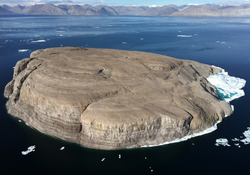This is a small, low-resolution photograph or photorealistic image capturing a tiny, rocky outcropping surrounded by the dark expanse of the ocean. The island, which is more of a solitary rock, features a slight, white sandy patch on its right side, suggesting a minuscule beach. Above the calm, yet dark waters, distant landmasses can be faintly seen on the horizon. There are unidentified floating objects around the island, potentially ice, hinting that the scene could be set in polar regions like Antarctica. Despite the pixelated and low-quality nature of the image, a strip of clear blue sky is visible above, adding a touch of color to the otherwise monochromatic scenery.